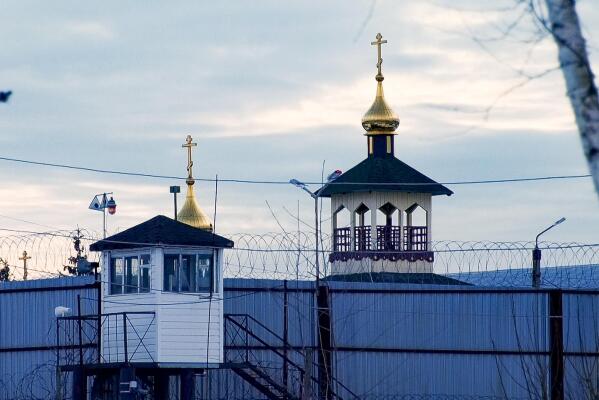This captivating image presents a church-like structure juxtaposed with elements that evoke a sense of confinement. Against a cloudy, grey sky, the scene is dominated by the tops of two chapels. The first, crowned with a golden bulb and cross, has the appearance of a gazebo with surrounding railings on a small elevated platform. The second, visible further back, shares a similar architectural crown with a cross. Dominating the foreground is a formidable metal fence, approximately 20 feet tall, topped with menacing barbed wire. Flanking this is a leafless tree and additional fencing—both wooden and metal—creating layers of barriers. In the background, a conspicuous watchtower, complete with a small building on a platform and windows all around, stands sentinel at the same height as the fence. Street lamps and power lines intersect the scene, and the entire composition is painted in shades of blue, white, tan, gold, and beige, adding to the intriguing and somewhat somber ambiance.